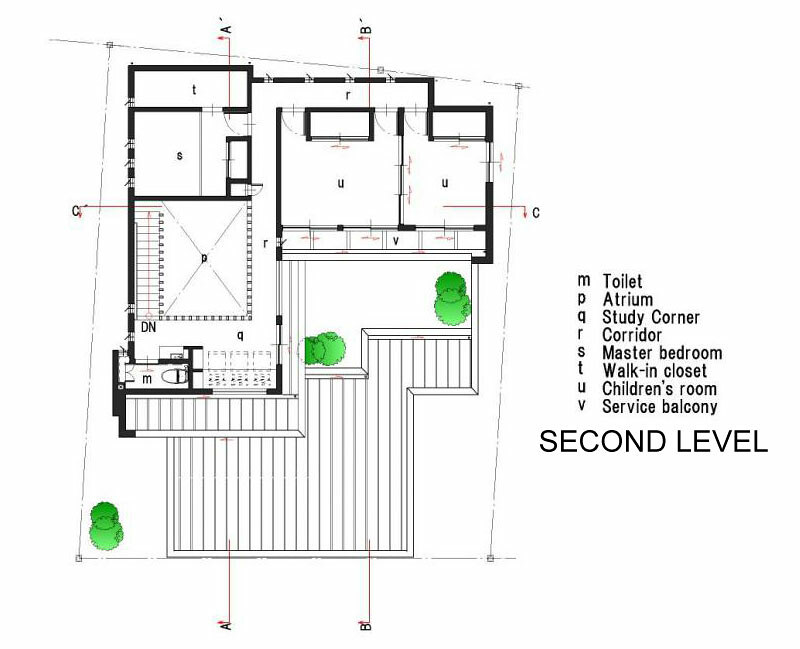The image is a detailed architectural blueprint of a house's second level, displayed on a white background. The design includes thick and thin black lines forming various rectangles and squares representing different rooms and areas within the house. Notably, there are labeled sections with capital letters indicating specific spaces: "M" for Toilet, "P" for Atrium, "Q" for Study Corner, "R" for Corridor, "S" for Master Bedroom, "T" for Walk-in Closet, "U" for Children's Room, and "V" for Service Balcony. A key on the right side of the blueprint explains these labels. Throughout the blueprint, green circles suggest the placement of flowers or bushes. The image is titled "Second Level" in prominent capital letters at the bottom.